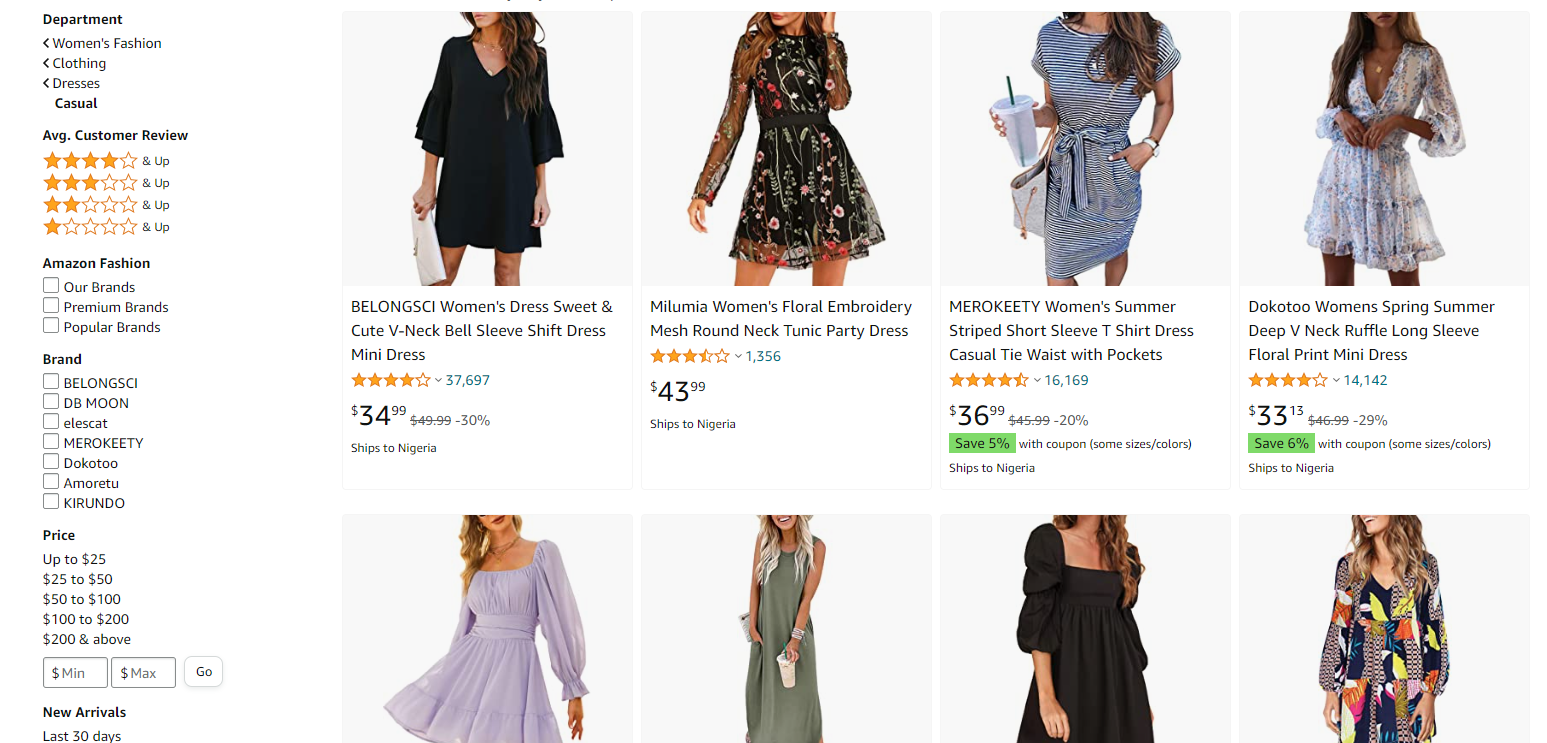A small screenshot from the Amazon.com website, likely the American version, showcases a selection of sundresses in the women's fashion section. Specifically, this appears to be the casual dresses category. The image features eight different models, each showcasing a unique dress. Several brand names are visible, including Belongsy, Malumia, Marokiti, and Dokutu, although the names suggest that this could be a version catered to another region, possibly India. The models, however, appear to be of Western descent. One prominently displayed dress is a deep V-neck ruffle long sleeve, priced around $31.15. Other dresses have similarly detailed names and prices, emphasizing a variety of casual fashion choices available on the site.